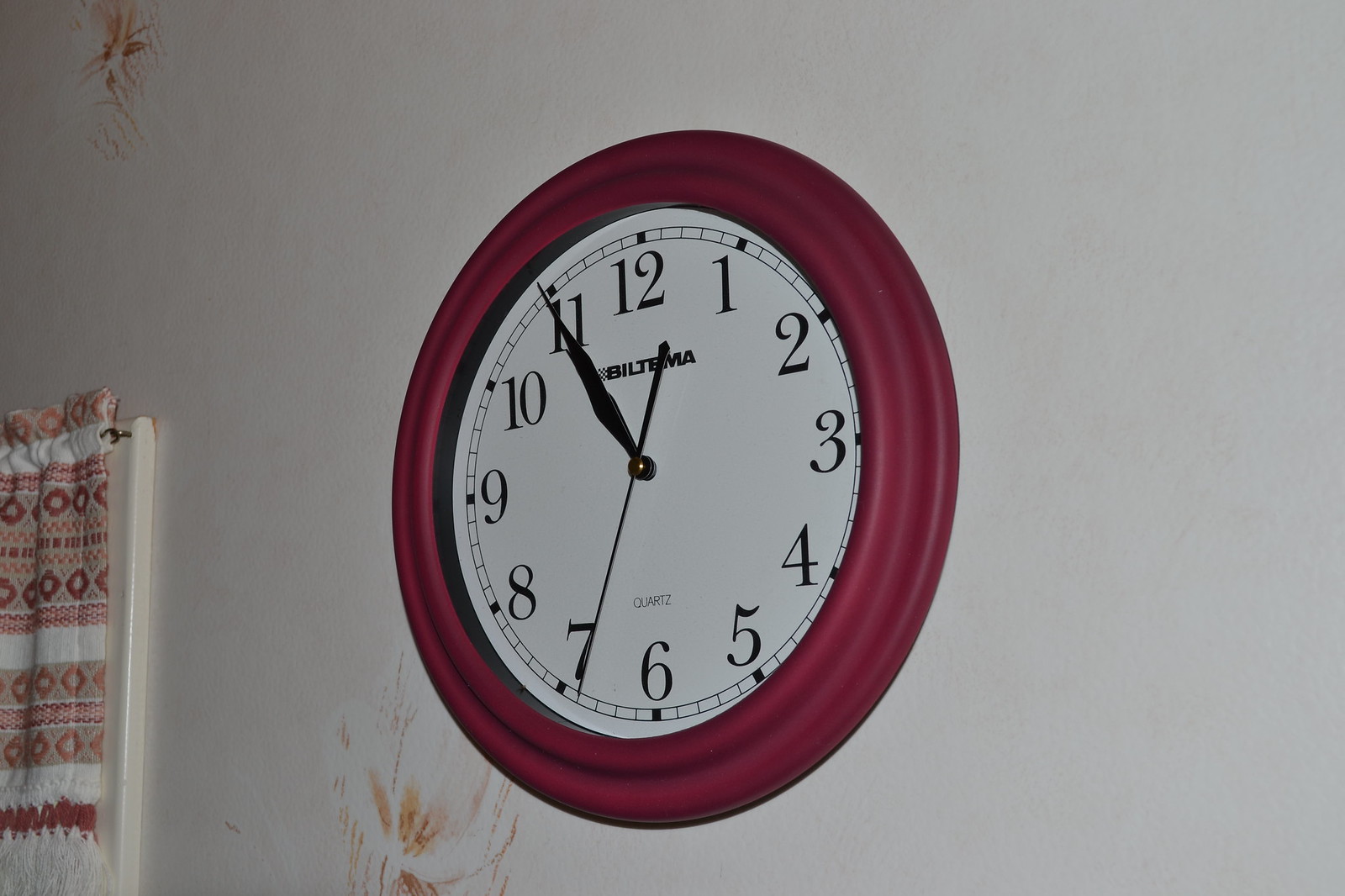The image showcases an interior wall that appears to be within someone's home, painted in a creamy white shade and partially in shadow. The wall features faint, spaced-out, light brown floral designs, possibly painted or drawn, adding a subtle decorative touch. Centrally positioned on the wall is a circular clock with a white face encased by a thick, dark red (maroon) border. The clock displays bold black numbers from 1 to 12, and it is approximately 10:54, with the minute hand about to reach the 7. The brand name "Biltema" is printed under the number 12, and the word "quartz" is located just above the 6. To the left of the clock, a partial view of a window frame is visible, adorned with a curtain that has a complex design featuring white, dark brown, and tan colors, reminiscent of a Native American pattern with geometric shapes such as squares and hexagons.